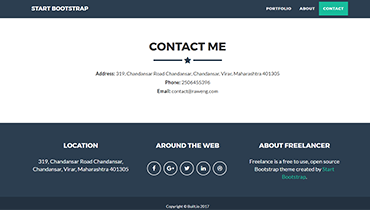At the top of the image, there is a black navigation bar with the text "Start Bootstrap" on the left and menu items "Portfolio" and "About" on the right. Also on the right side of the navigation bar, there is a green button labeled "Contact." Below the navigation bar, the background transitions to white. Prominently displayed in the center of this section is the text "CONTACT ME" in bold, black, capital letters. This text is flanked on either side by horizontal lines with a star in the middle. 

Below "CONTACT ME," there are several sections with the following headings: "Address," "Phone," and "Email." Under each heading, the respective information is displayed but appears blurry and illegible.

Further down, there is another black box containing more blurred text starting with "Location," followed by numerical sequences such as "319" and "401 305." 

Finally, at the bottom, there is a section titled "Around the Web." Under this, it briefly describes "Freelancer" as a free service with additional blurred, unreadable text, mentioning it is created by an unspecified individual.